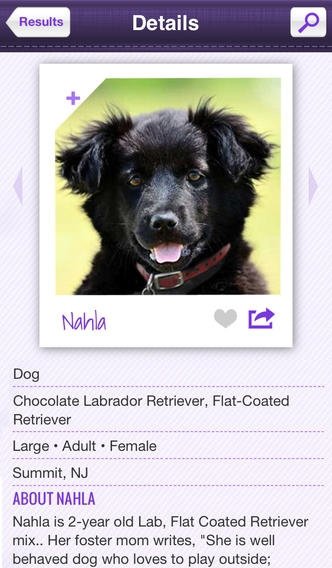In this detailed image, a rich, dark purple background serves as the canvas. On the left side, bright blue and purple letters form a square box with sharp left edges and a pristine white background. In the center section, white lettering spells out "Details" clearly. Adjacent to this, a box with a white background and a purple magnifying glass illustration seamlessly fits in. 

At the bottom, the image features a subtly mixed light purple and white lined backdrop. Two purple arrows, one pointing left and the other right, flank the center, where a white-outlined picture of a black dog with a brown leather collar is displayed. Below the picture, the name "Nala" is inscribed on the left. A purple plus sign adorns the top left corner of this frame while the bottom right corner has a grey heart and a purple arrow pointing to the right, partially encircled by a half square. 

Further down, in black font against the backdrop, the text lists:
- "Dog" followed by a grey dotted line
- "Chocolate Labrador Retriever, Flat-Coated Retriever" followed by another grey dotted line
- Another chain of words saying "Adult · Female" followed by a dotted line
- "Summit, New Jersey" again followed by a dotted line
- "About Nala" highlighted in purple

The description continues, noting that Nala is "a two-year-old Lab, Flat-Coated Retriever mix… Her foster mom writes, she is a well-behaved dog who loves to play outside."

Encasing all of this, there is a green background that brilliantly contrasts the overall purple theme and highlights the black dog, Nala.